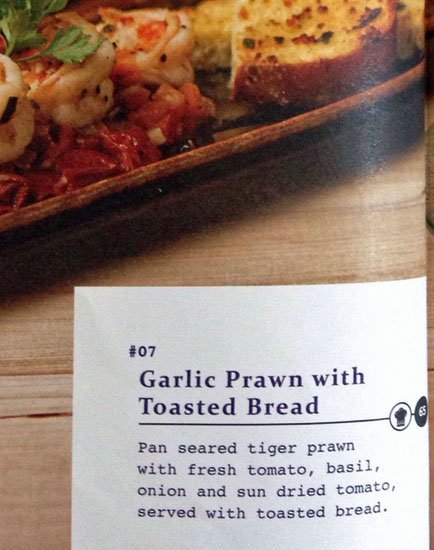This is a detailed close-up photograph of a recipe page from a magazine or book. The page features a vibrant image of a culinary dish served in a wooden oval dish, placed on a wooden table. The dish consists of pan-seared tiger prawns accompanied by fresh tomatoes, basil, onions, and sun-dried tomatoes, all served with toasted bread. The food is artistically arranged, with the prawns on the left and the bread on the right, garnished with green leaves and additional ingredients. Situated in the bottom part of the image, there's a large white rectangular box containing black or dark purple text. The text reads: "Ash 07 Garlic Prawn with Toasted Bread - Pan-seared tiger prawn with fresh tomato, basil, onion, and sun-dried tomato served with toasted bread." This box adds a brief but precise description of the dish, aligning with the visual presentation above it. The page appears slightly curved on the right side, adding a subtle dynamic element to the photograph.